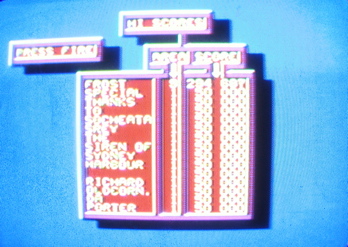Caption: 

This image captures the high score screen of a vintage 1980s computer game. The layout is landscape-oriented with a wider-than-tall aspect ratio. The background is predominantly blue, featuring a lighter white circular gradient in the center. Multiple coral-colored boxes with purple outlines populate the screen. 

In the upper left corner, a large rectangle displays the text "Press Fire." Above this, a header reads "High Scores," connected by a small line segment to another text box below. The left header, though unclear, is juxtaposed with "Score" on the right, followed by a down arrow indicating the list that follows. Two columns of numerical scores are prominently displayed.

Separating these columns are purple and white divider lines, to the right of which a list of names is visible. These names, including "Frost," "Special," "Thanks," "Richard," and "Porter," likely represent players or contributors who have achieved high scores or special recognition within the game. The nostalgic graphics evoke the iconic, pixelated style typical of classic computer games from the 1980s.